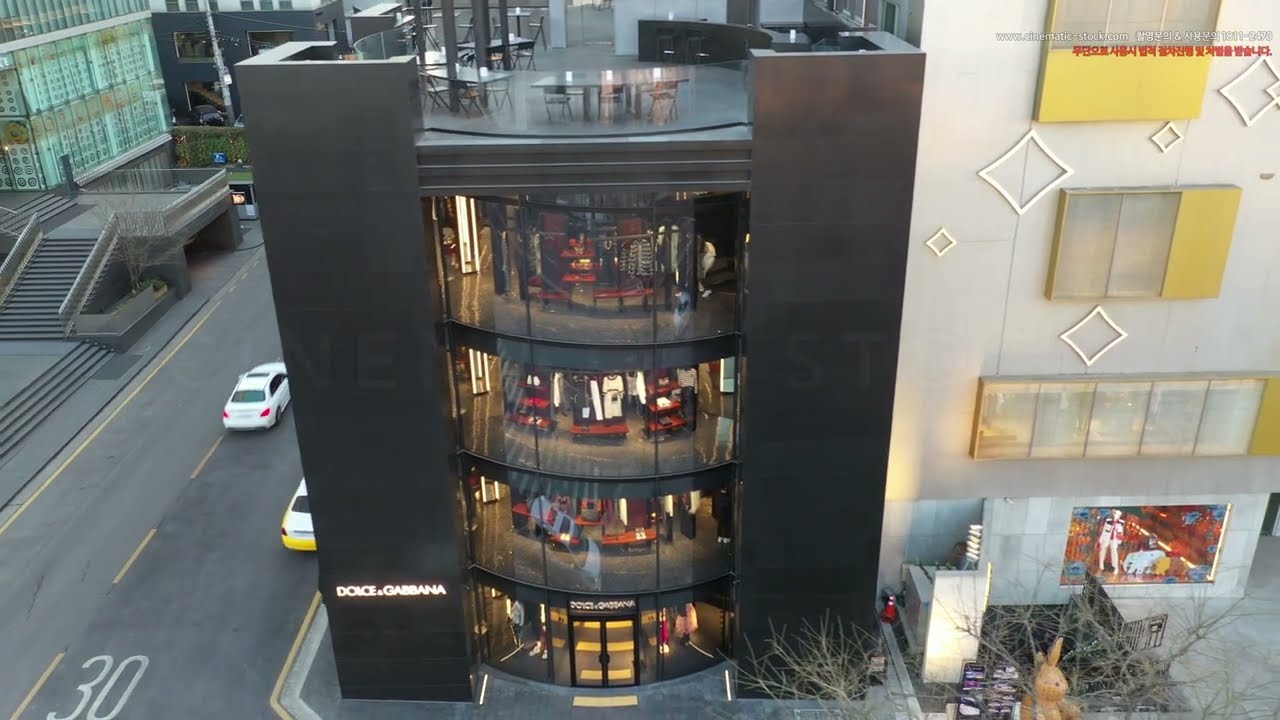The image depicts an urban street scene with a prominent focus on two distinct buildings. On the right side, the primary building is a sleek, four-story Dolce & Gabbana store featuring two prominent black columns on each side and convex, oval-shaped, glass-panelled walls that allow visibility into the interior. At the ground level, the Dolce & Gabbana logo is displayed above a double glass entry door, and the rooftop area is set up as an outdoor café with tables and chairs. Adjacent to this structure, further to the right, stands a four-story white building. This building's facade is enhanced with diamond-shaped yellow accents, and its ground floor showcases a window with a mannequin and other interior merchandise. On the left side of the image, a road marked with yellow stripes features two sedans traveling away from the viewer, underscoring the dynamic, city life ambiance of the scene.